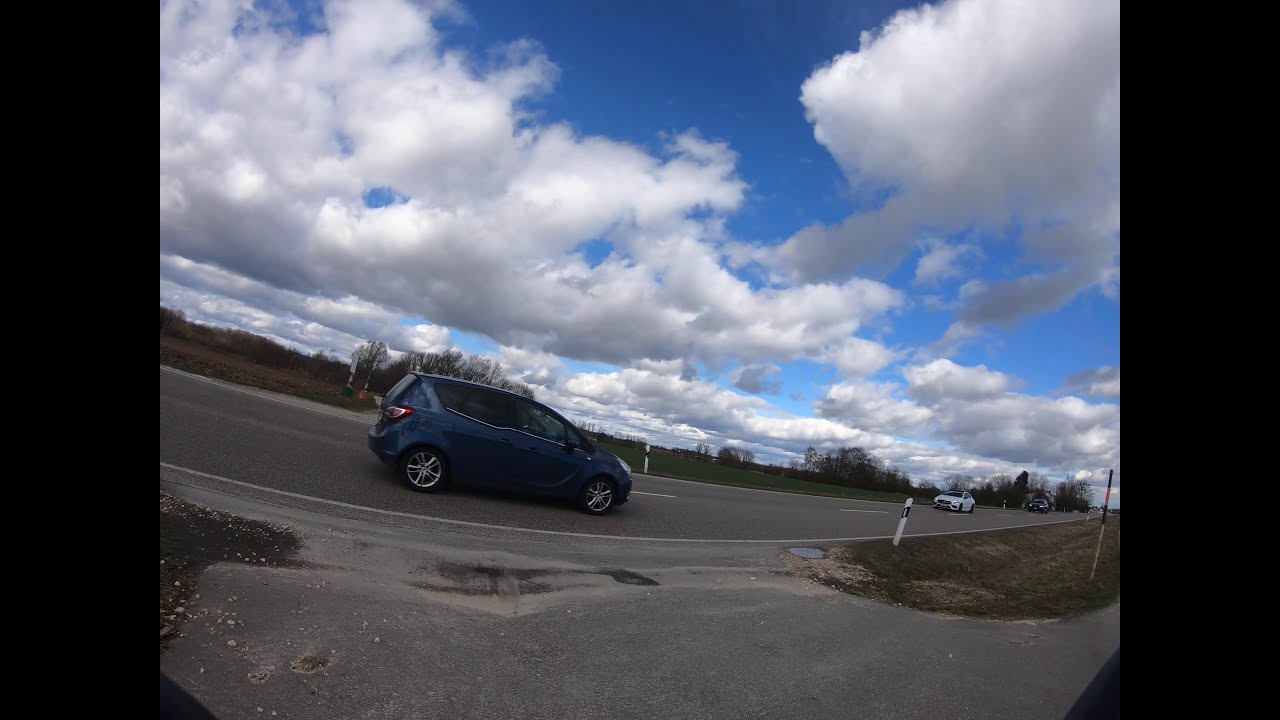In the image, an outdoor daytime scene unfolds with a two-lane road extending horizontally. The road, made of light gray asphalt, is marked by a white center line and flanked by two small white pillars with black stripes, indicating an intersection. The sky above is a vibrant mix of dark and light blue, dotted with various white and gray clouds. 

From the vantage point on the shoulder of the road, the closest vehicle is a dark blue subcompact car with silver rims, moving left to right. In the distance, on the far side of the road, a white sedan is seen approaching, followed by a black sedan further back. The backdrop features trees and some vegetation or a field, contributing to the serene roadside atmosphere. The image appears slightly distorted with a fisheye effect, suggesting it might have been captured with a smartphone camera, and it is subtly tilted, higher on the left than on the right. The scene hints at midday lighting, with sunlight illuminating the landscape.